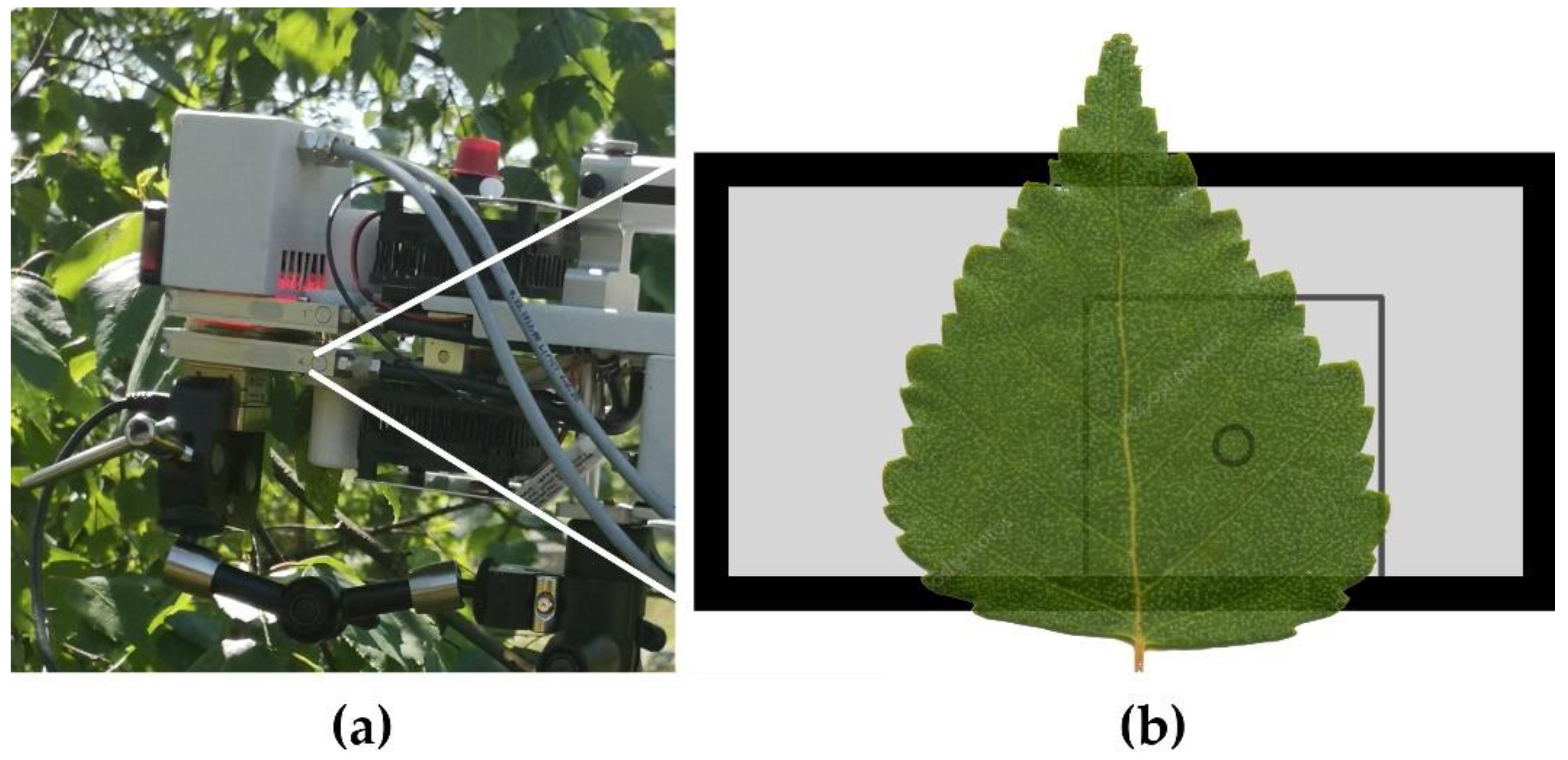The image consists of two side-by-side photos labeled with black letters in parentheses: the left photo labeled (A) and the right photo labeled (B). 

Underneath image (A), there is a white box featuring various scientific equipment amidst leafy green branches, indicating it is set up outdoors. This equipment primarily comprises a central square structure housing what appears to be a lens or surveillance device, possibly for observing or recording. To the left of this square, there is a gray box with wires extending from the top downwards and additional black equipment below it, including gray bars and more cords exiting the setup and moving out of the image frame. The apparatus seems complex and is crafted from various materials including white metal and black components, suggesting a purpose related to scientific measurements or observations.

Image (B) on the right, which is labeled similarly with a (B) underneath, presents an enlarged section seemingly linked to the device shown in image (A). In this part, there is a horizontal rectangle outlined in black, filled with light gray coloring. Inside this rectangle, there is an outlined square containing a circle, upon which lies an image of a green, semi-transparent leaf with a short stem and a pointed tip that slightly extends outside the rectangle at the top and bottom. This setup seems to be part of the scientific process, possibly measuring or analyzing some properties of the leaf.